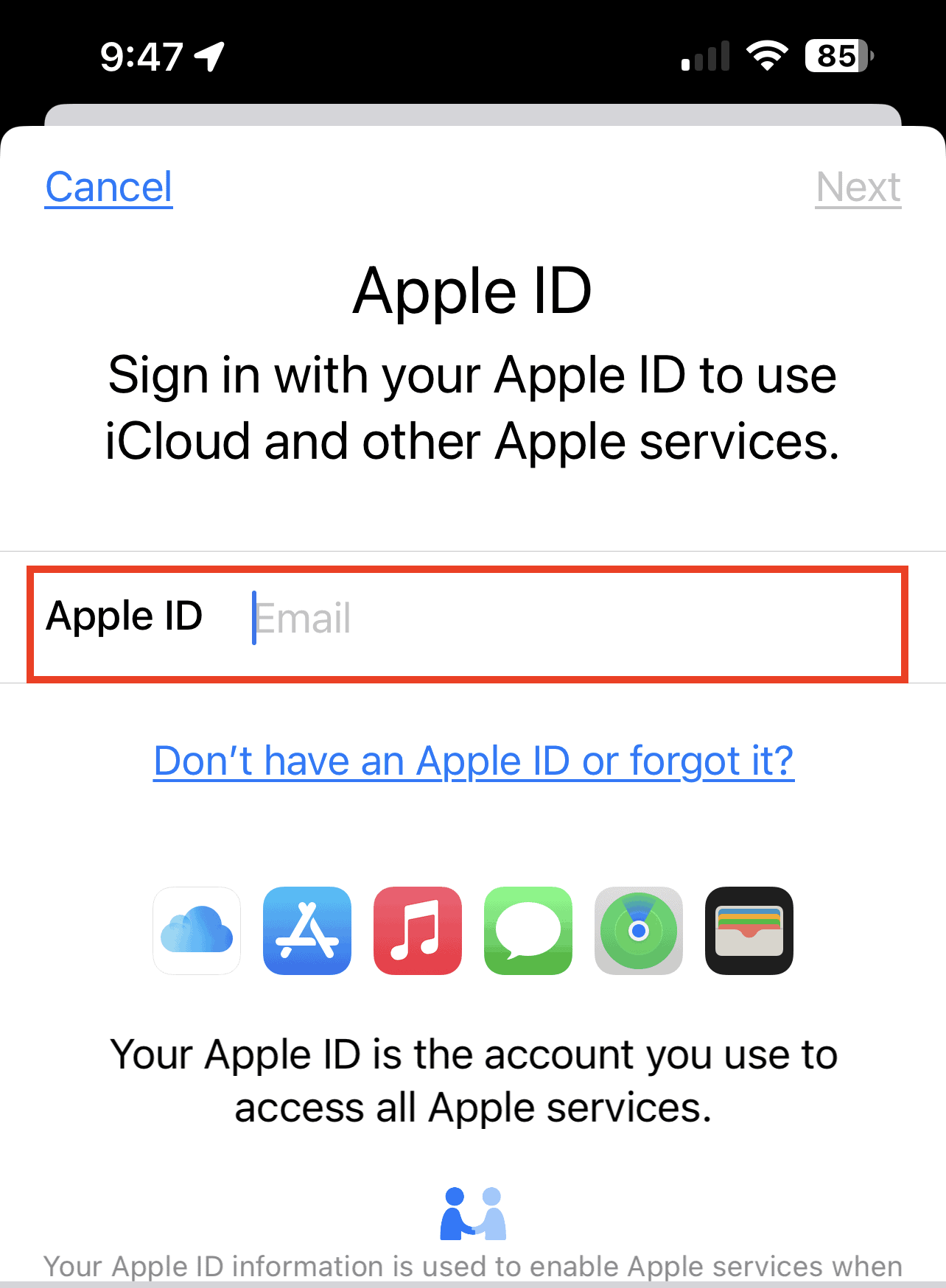The image showcases an Apple device screen, likely an iPhone or iPad. At the top of the screen, the time is displayed as 9:47 AM, with a strong Wi-Fi signal indicator. Beside the Wi-Fi icon, there's a number '85,' potentially indicating signal strength or battery percentage. In the top left corner, a blue "Cancel" option is visible, while on the right, a grey "Next" button is present.

Prominently centered at the top is a heading: "Apple ID." Below it is a prompt: "Sign in with your Apple ID to use iCloud and other Apple services." A red-highlighted box contains a prompt for the Apple ID email, with a cursor ready for typing. Beneath the Apple ID field, there's a label indicating "Email." Further down, a link states "Don’t have an Apple ID or forgot it?" followed by various icons representing payment, music, texting, and chatting services.

At the very bottom of the screen, two character icons are displayed in the center; one is a darker blue, and the other is a lighter blue, with both engaging in a handshake. This symbolic image reinforces the collaborative and integrated nature of Apple services.